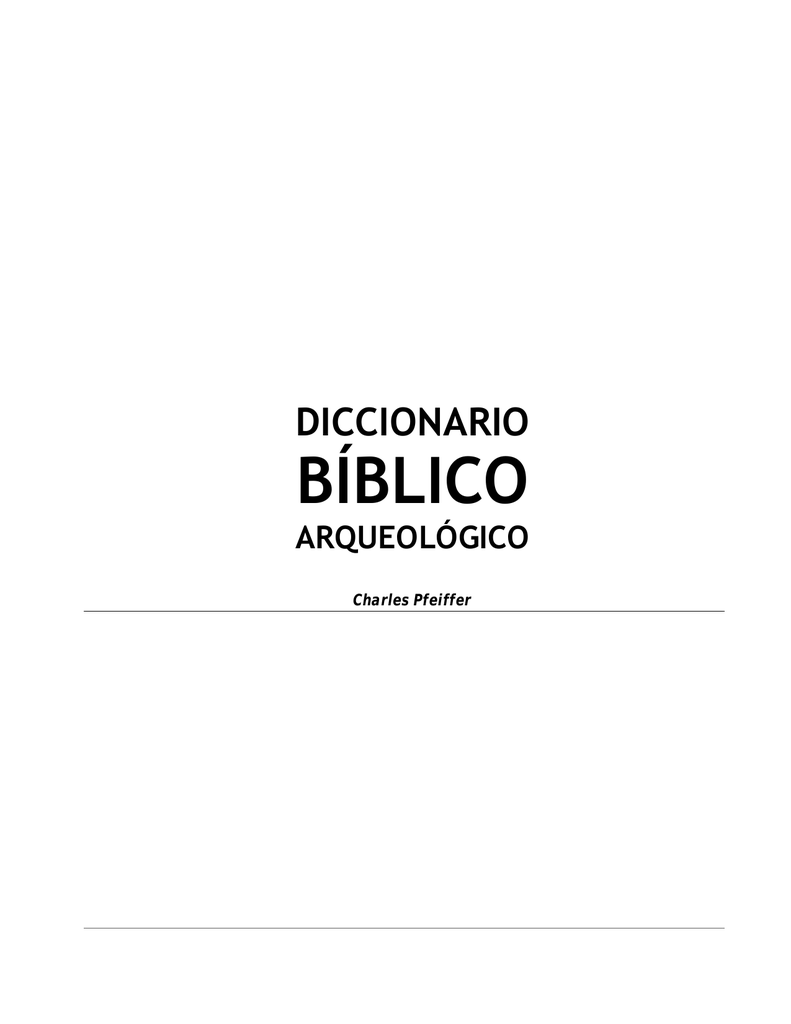The image features an elegantly simple design against a pure white background, resembling a book cover or the first page of a document. The central text is in Spanish and formatted in four lines. The top line reads "Diccionario" in a medium-sized font, followed by "Bíblico" in a larger font, making it the most prominent word despite being the shortest. The third line shows "Arqueológico" in a medium-small font. Below these, in the smallest text, is the name "Charles Pfeiffer." A thin horizontal line underlines the author's name, and there is another thin horizontal line at the bottom of the image, creating a balanced visual structure. There are no objects, additional text, or decorative elements, emphasizing the stark, professional aesthetic of the cover.